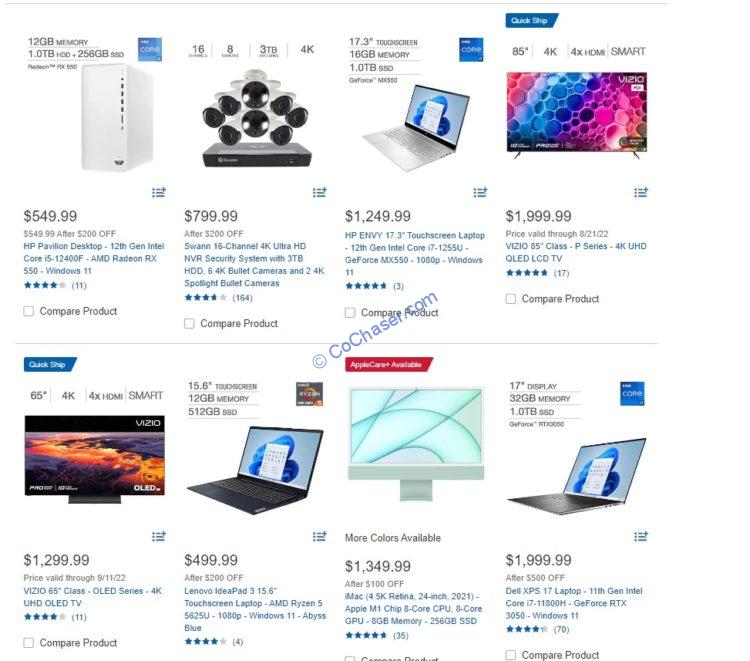In this image, set against a solid white background, there are several items for sale prominently displayed. 

**Top Left**: Features technical specifications including a 12 GB memory and a 1.0 TB HDD, with an additional mention of 25.8 GB. Adjacent to these specs is a white rectangular object that appears to be part of the product display.

**To the Right**: A large price tag that reads "$799.99 after $200 off" is prominently displayed. Below this, a detailed description highlights the "SWAN 16 channel 4K Ultra HD NVR security system" which comes with a 3 TB HDD, 6 4K bullet cameras, and 2 4K spotlight bullet cameras. This product boasts an almost 4-star rating based on 164 reviews.

**Lower Left**: A black monitor is displayed with the price "$1,299.99," valid through September 11, 2022. Below this, a detailed description reads "Vizio 65-inch class LED series 4K UHD OLED TV," which has received a 4-star rating from 11 reviews.

Overall, the items range from high-performance memory and HDDs to advanced security systems and top-tier televisions, each boasting notable discounts and consumer ratings.